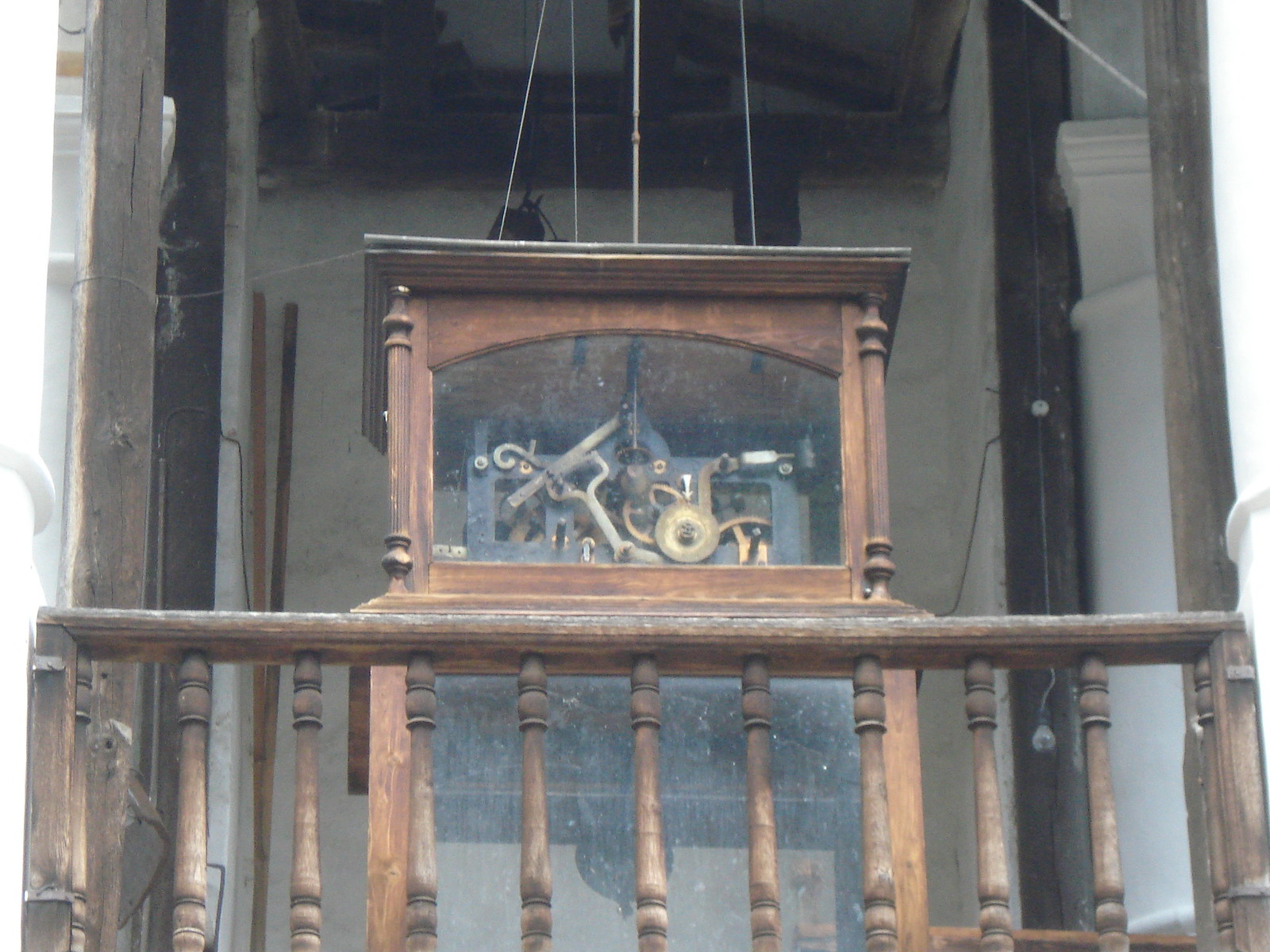The image displays an intricate mechanical mechanism housed within an ornate wooden and glass display case. The case, featuring clear walls that reveal the complex machinery inside, is set against a white wall with prominent wooden beams on either side, creating the appearance of an old, stuccoed building. The mechanism itself comprises a black metal frame with numerous brass components, including gears, pipes, levers, and linkages, suggesting it might be a form of a clock. Three taut cables and a vertical rod extend from the top, interacting with the elements within. In the foreground, the display case is situated behind an elaborate wooden balcony railing with turned uprights and a profiled top, adding to the scene's architectural charm.